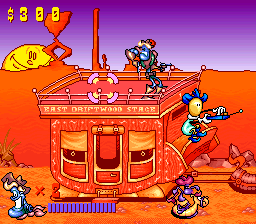In this pixelated scene reminiscent of an old video game, an orange-shaped horse-drawn carriage is set against the backdrop of a barren desert. The sky, a deep purple, showcases a setting sun with a whimsical smile. The carriage, detailed with a door and two side windows, has a character standing on its roof, brandishing a gun. This character surveys the surroundings with a vigilant stance. Seated in the driver’s seat is a character with blue hair, clutching a blue remote with an antenna. Below the carriage, a rider atop a snail-like creature adds to the surreal ambiance. To the right, a female character in a blue dress walks away from the scene, adding a touch of mystery to this curious tableau.